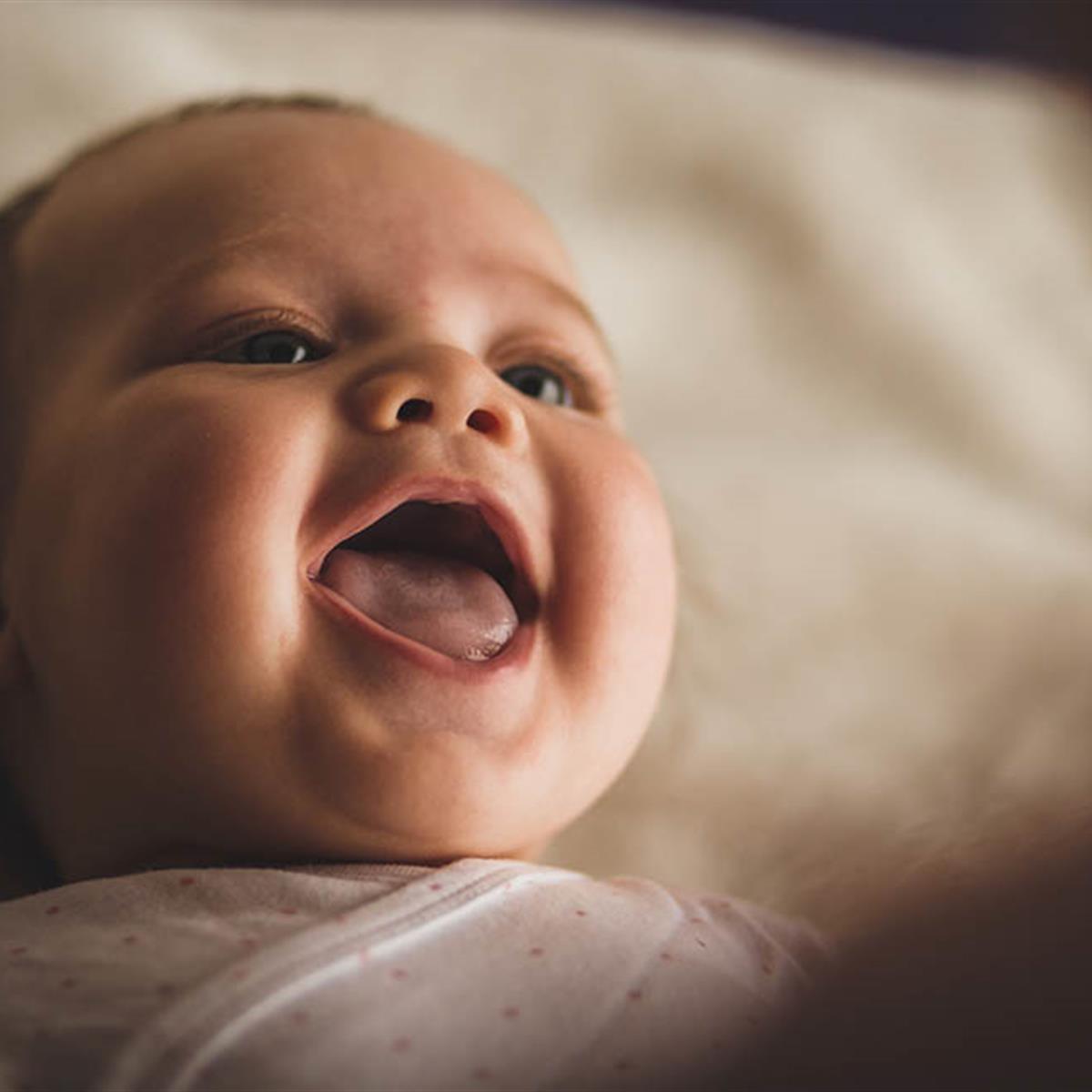This is a detailed color photograph of a joyous infant lying on their back in what appears to be a crib or on a pillow, with a predominantly white, slightly out-of-focus background. The image is square in format, with the baby positioned on the left side, captured from the top of the head to just below the chest. The baby is wearing a white outfit adorned with faint red or pink dots, resembling a pajama or gown that crisscrosses in the front. The baby's face, which is the focal point of the image, exhibits a very happy expression with an open mouth, visible tongue, and no teeth. The baby is gazing slightly off to the side of the camera, showcasing light skin, light brown hair, and light blue eyes. The background includes white linen with some folds, suggesting a blanket or crib setting. On the right side of the frame, a blurry dark area, possibly someone's finger or head, intrudes into the image.